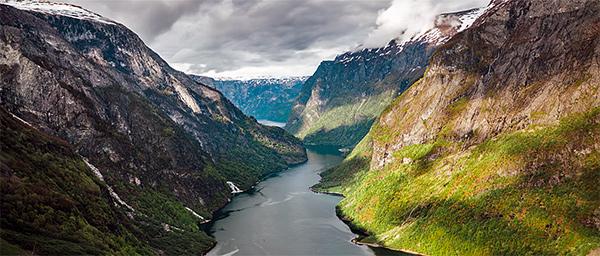This captivating photograph features a sweeping landscape of a mountain valley with a wide, serene river running through it. The valley is nestled between two formidable mountain ranges, each boasting a rich tapestry of colors and textures. To the left, the mountain is predominantly rocky with dark blues and grays, gradually transitioning to greenery and shrubbery at its base. As the altitude increases, patches of snow become visible, adding a stark contrast to the rocky surface. On the right, the sun illuminates the mountainside, highlighting its lush green vegetation and distinct orange and brown hues. The slopes here are steeper and more rugged, with visible moss and foliage. In the distant background, additional rocky, snow-capped peaks can be seen under a canopy of dark gray clouds. The river itself appears calm and wide from this vantage point, with subtle ripples hinting at an underlying current, elegantly bisecting the tranquil yet majestic landscape.